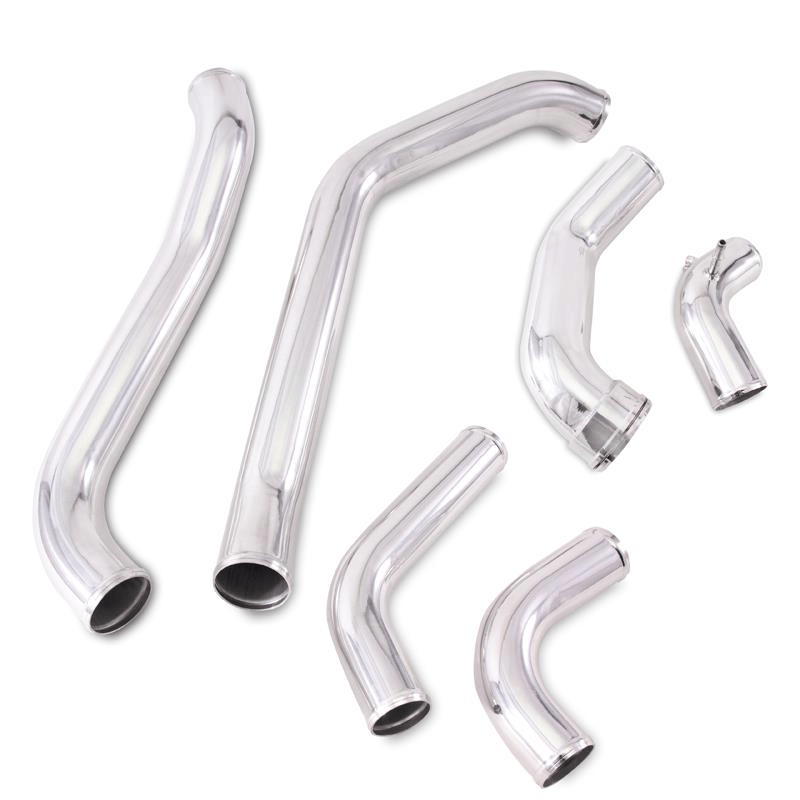The image features a collection of polished, shiny stainless steel pipes arranged against a white background. There are six pipes in total, each varying in size and shape. The leftmost pipe curves gently at both ends, resembling a subtle backward 'S'. To its right, a pipe mimics the shape of a faucet, curving sharply at the top. Further to the right, there are four shorter pipes. On the lower right, one pipe features a single, smooth L-shaped curve, while another forms a nearly complete 'C' shape. The remaining two pipes, one located at the upper right corner, also display slight curves. Each pipe has an open end, giving a glimpse of the inner surface and adding depth to the composition.